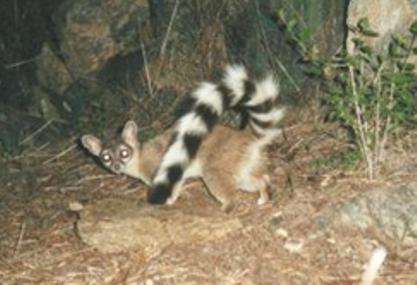The photograph, taken at night, captures a wild animal illuminated by a camera flash, making its eyes appear as glowing white bulbs. The creature, which resembles a Tasmanian devil or perhaps a species related to a raccoon, features a striking black and white ringed tail. The tail alternates between black and white rings, ending in a black tip. The animal appears to be walking towards the upper left corner of the frame while looking back at the camera, revealing its brown fur with white underbelly and bar-like white markings on its left side. Surrounding the animal are elements of its natural habitat: green leaves on a small shrub to the right, a tall tree trunk in the background, and the ground beneath it strewn with rocks and weathered brown leaves that hint at out-of-season grass.